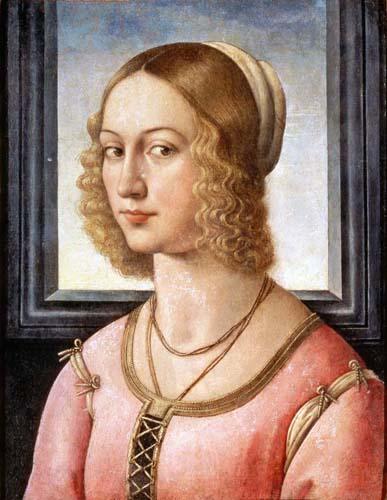This detailed portrait, reminiscent of the style of masters like Da Vinci or Rembrandt, depicts a woman with golden blonde, neck-length hair that is straight on top and curly towards the bottom, some strands framing the side of her face. She wears a white cap at the back of her head. Her expression has a Mona Lisa-like serenity, with hazel or light brown eyes looking slightly down and to the left, while her face and body are turned to the right.

She is dressed in a pink garment with gold trimmings, featuring crisscross strings up the front, and adorned with ribbons tied at the sleeves. Beneath, she seems to be wearing a darker shirt. Around her neck, she wears a gold necklace, which appears to be folded over twice.

The background includes a black-framed window, part of which is visible behind her, revealing a blue sky with clouds towards the upper half and a whiteness towards the lower half. The black window frame contrasts with the bright, airy scene outside, adding a sense of depth to the painting.